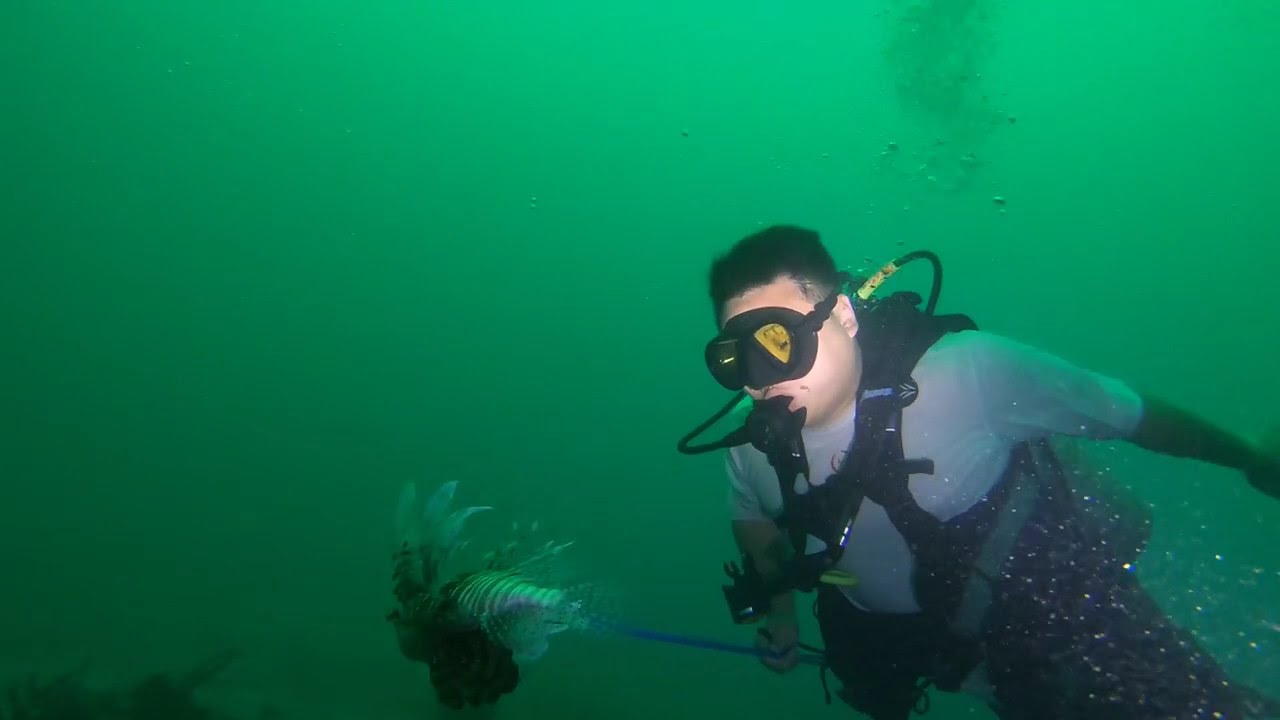An underwater scene features a scuba diver equipped with a mask, a breathing apparatus, and an oxygen tank. He is wearing a white t-shirt rather than a typical diving suit and dark-colored bottoms. His black hair and slight mustache are visible, while his goggles have a yellow tint. Strapped around his shoulders, chest, and waist are black gear and tubes leading to his mouthpiece. The water around him is a murky greenish-blue, creating a dimly lit, hard-to-see background. The diver has just speared a striped fish with slightly transparent, frilly fins. Bubbles from his equipment ascend through the water, adding to the dynamic underwater scene.